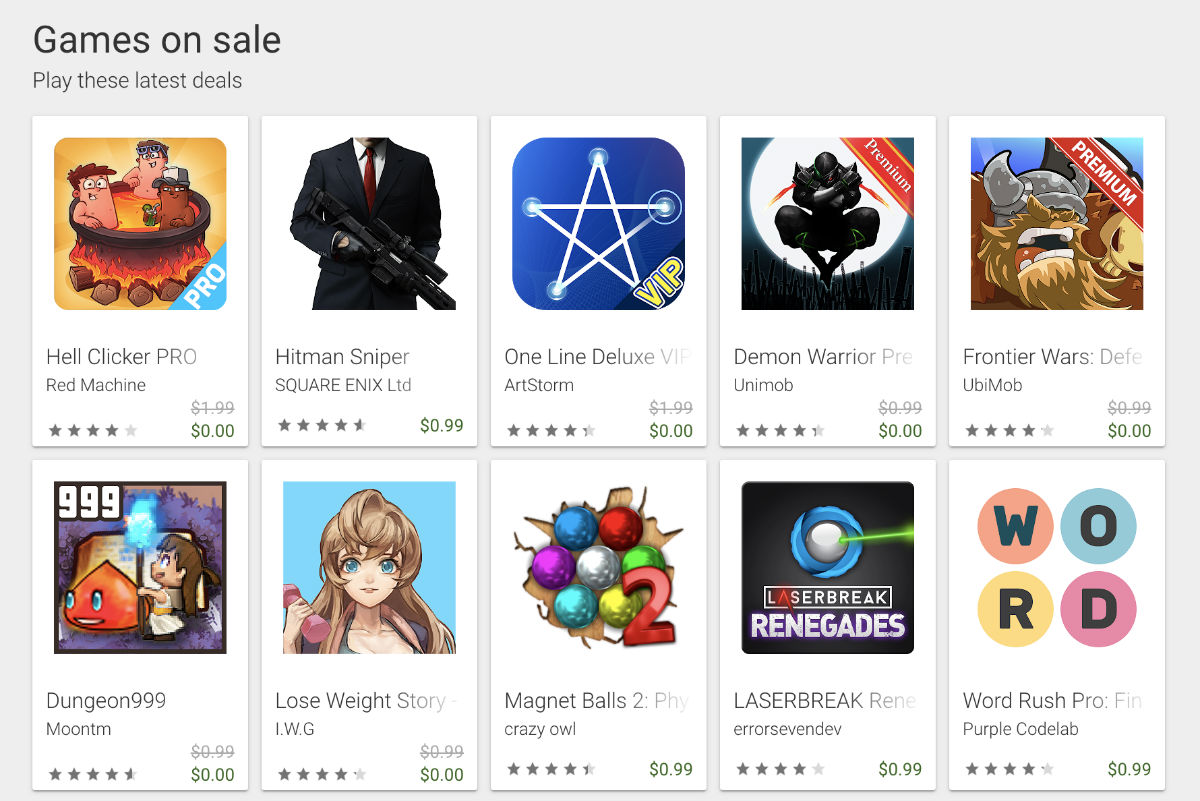The image depicts a layout of apps available in the Google Play Store, specifically showcasing "Games on Sale." The promotional banner reads, "Play these latest deals," and below it are two rows, each containing five game icons. The featured games are: Hell Clicker Pro, Hitman Sniper, One Line Deluxe, Demon Warrior, Frontier Wars, Dungeon 999, Lose Weight Story, Magnet Balls 2, Laser Break, and Word Rush Pro. 

The prices of the games are significantly discounted, with some being offered for free. For instance, a game originally priced at $1.99 now shows as $0, and one that was $0.99 is also marked down. The visual design of the game icons is diverse: one features an anime character, another depicts a hitman with a sniper rifle, and yet another shows a Viking with helmet horns. The style ranges from realistic to cartoonish, appealing to a wide array of gaming preferences.